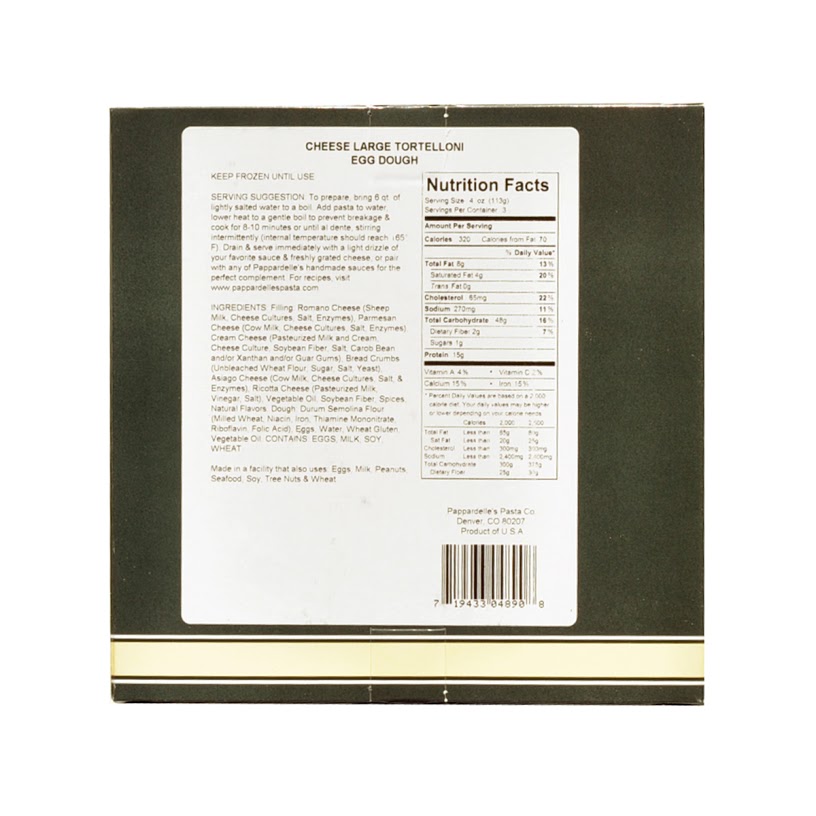This rectangular image features a nutrition facts label for Cheese Large Tortellini Egg Dough prominently displayed against a dark green background. The label itself is a large white rectangle with text in black and green. At the top, it states "Cheese Large Tortellini Egg Dough." Beneath this, it offers detailed serving instructions: "Keep frozen until use. To prepare, bring six quarts of lightly salted water to a boil, add pasta, lower heat to a gentle boil to prevent breaking, and cook for eight to ten minutes or until al dente. Drain and serve immediately with a light drizzle of your favorite sauce and fresh grated cheese, or pair with any of Pepper Dell's handmade sauces for the perfect complement. For recipes, visit www.pepperdellipasta.com."

The left side of the label lists all the ingredients, along with an allergy warning that the product is made in a facility that also processes eggs, milk, protein, seafood, soy, tree nuts, and water. The right side of the label displays the Nutrition Facts, detailing information like calories, total fat, cholesterol, total carbohydrates, and a breakdown of vitamins.

Below the Nutrition Facts section, there is a UPC code, followed by the text: "Product of USA. Prepared by Pepper Dell Pasta Company, Denver, Colorado." A yellow stripe with green lines runs horizontally along the bottom of the image, adding a contrasting accent to the overall design.